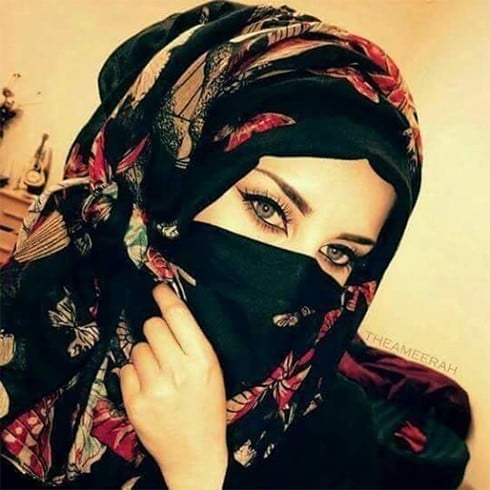The image portrays a head-and-shoulders portrait of a woman adorned in a burqa with an intricate and pleasant floral design, predominantly black with accents of red, yellow, brown, green, and white. Her eyes, which are a striking blue or hazel, and her meticulously lined eyebrows and long eyelashes, possibly enhanced with makeup, are prominently visible. The burqa covers her mouth and most of her face, revealing only her forehead, eyes, and the bridge of her nose. Her hand, which appears slightly odd with one long finger and three shorter ones possibly indicating an AI-generated image, is delicately holding the fabric across her face. The woman gazes directly into the camera with a slight angular tilt to her pose. The light brown background harmonizes with her skin tone, and subtle text on her shoulder reads "the Amira." The setting appears to be a bedroom, suggested by the beige walls and a dresser in the background, hinting at a candid or intimate moment captured in a homely environment.